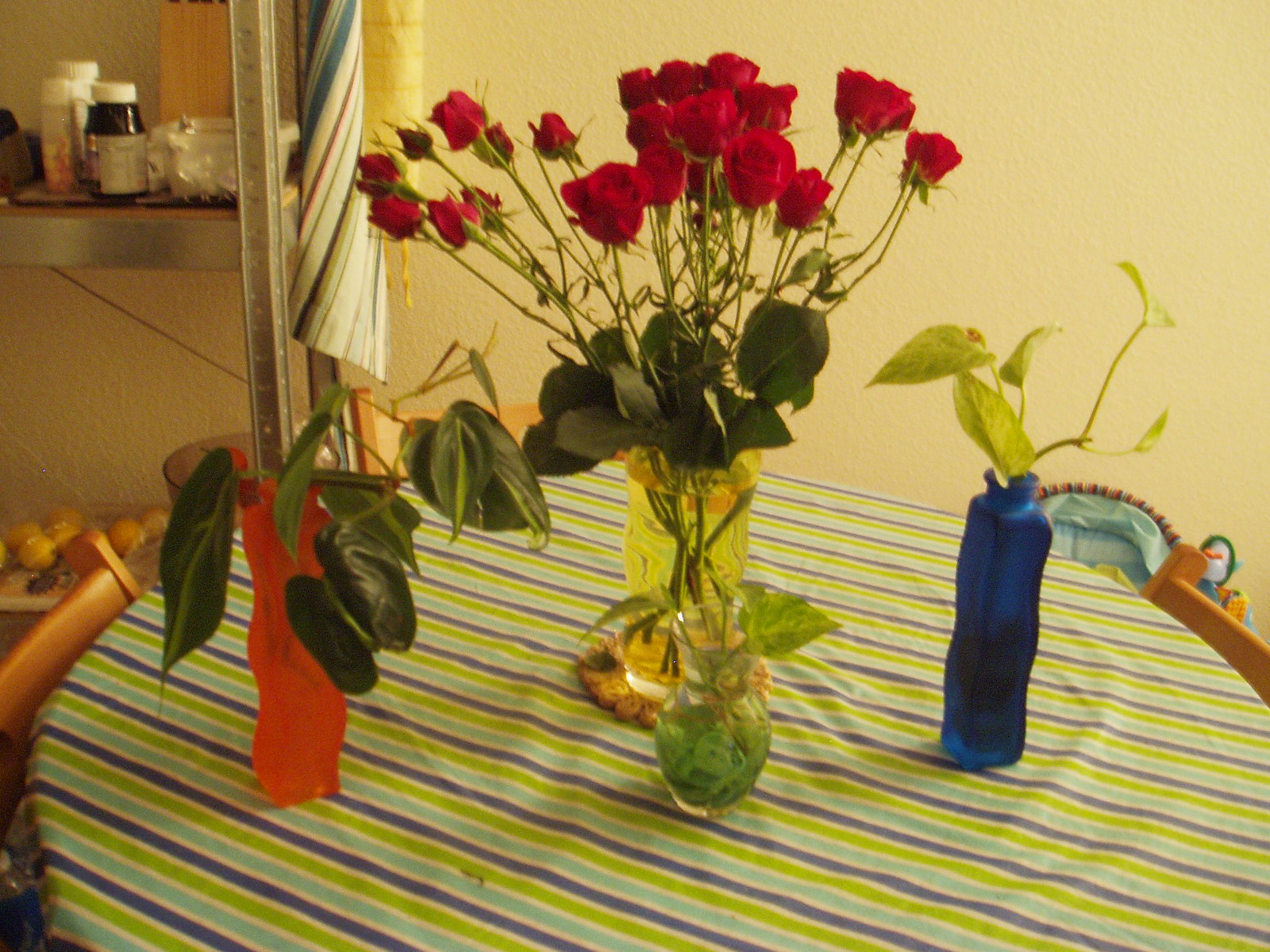This photograph features a round table draped with a tablecloth displaying horizontal stripes in shades of green, teal, light blue, and dark purple. Resting on the table are several vases of varying colors and plant arrangements. Centered in the composition is a clear yellow vase containing red roses with green leaves at the base. To the left of this central vase is a reddish-orange planter housing ivy, and to the right is a blue vertical vase, also containing ivy.

Behind the table, the yellow wall serves as a background to a silver, metal shelf stocked with various bottles, which appear to be either medication or plant nutrients. Adding more texture to the scene, a folded umbrella is perched in the corner, partially visible. The overall ambiance of the photograph is a vibrant interplay of colors and natural elements, framed by the distinct yellow hue of the background wall.